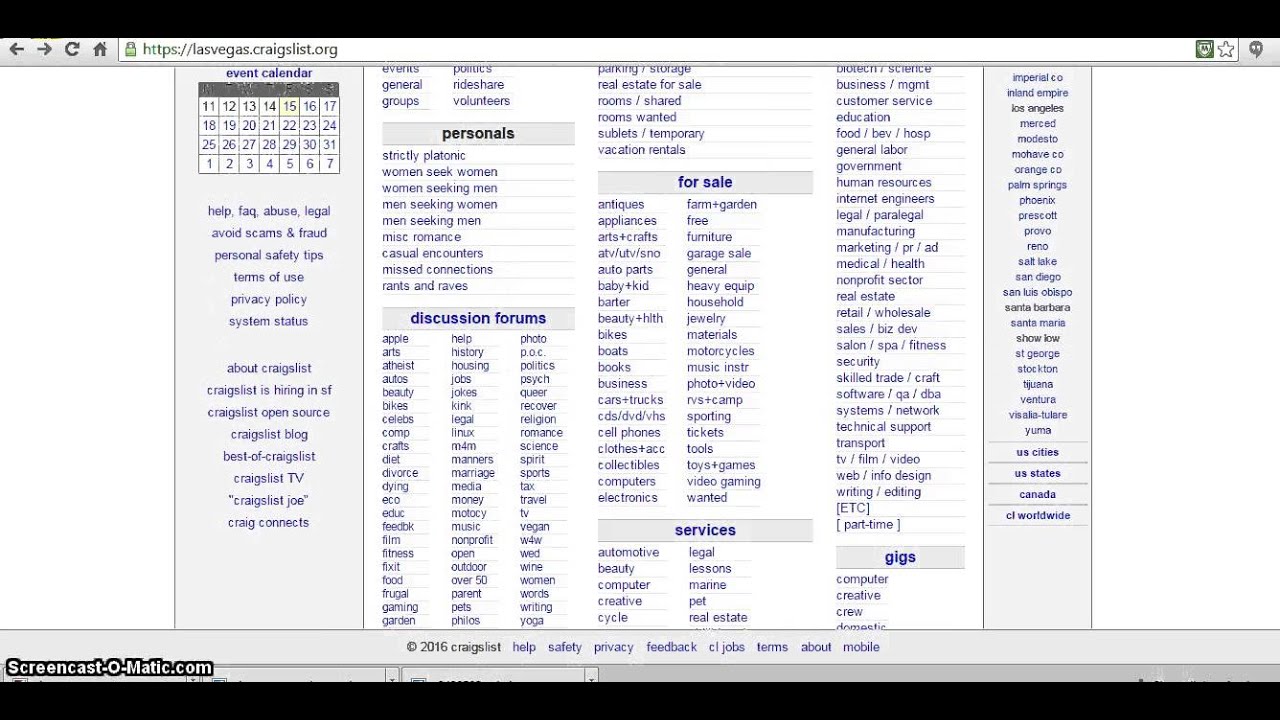The image depicts a web browser window showing the Craigslist website for Las Vegas. The address bar at the top indicates the URL as "https://lasvegas.craigslist.org." Below the address bar, the page features an event calendar. Notably, the calendar layout is unorthodox: the first row of dates displays "11 - 17," followed by "18 - 24" on the second row, "25 - 31" on the third, and "1 - 7" on the fourth row.

To the right of the calendar, a list of categorized sections is displayed. The "Personals" section is listed at the top, followed by "Discussion Forums." Below these, there are further categories such as "For Sale" and "Services." The "Services" category includes an extensive list of offerings, such as education, manufacturing, security, and sales.

Towards the far right, the "Gigs" section is highlighted in blue, featuring options like computer gigs and creative gigs. The rightmost column continues with vertical text listings, which include search options for "US Cities," "US States," and "Canada."